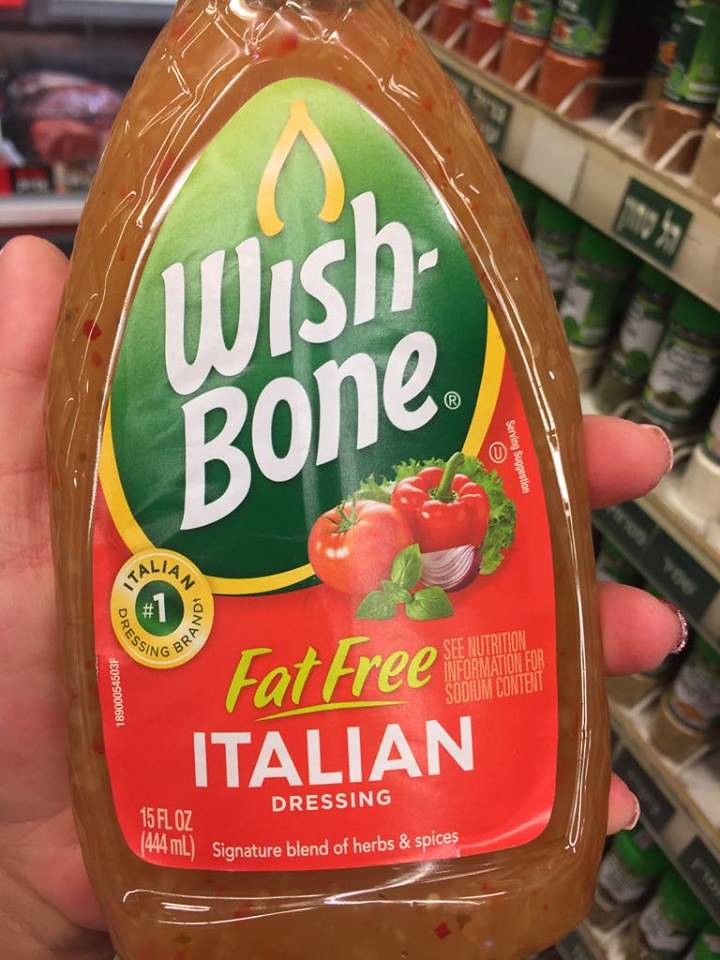This detailed close-up photograph features a plastic bottle of Wishbone fat-free Italian dressing, held up by a hand, likely a woman's, with the thumb and tips of the fingers visible around the back of the bottle. The bottle is clear, showcasing the brown-orange liquid inside speckled with red flakes of spices, suggesting a lighter-than-usual Italian dressing.

The label on the bottle has a distinctive design, starting at the top with a green background and white lettering that reads "Wishbone," accompanied by a yellow Wishbone logo above it. Below the green section, the background changes to red with "fat-free" in bold yellow text. The label continues with "Italian dressing" in white text, highlighting the fact that this is the #1 dressing brand in Italy.

The bottom part of the label features vibrant images of fresh ingredients: a red tomato, a red pepper, some lettuce, basil, and a piece of onion. The label also mentions "signature blend of herbs and spices" and includes a prompt to check the nutrition information for sodium content. The setting of the photograph appears to be in a supermarket, likely in the spice section, and there is a possibility that the location is Israel or another area where Hebrew is spoken, inferred from visible signages in the background.